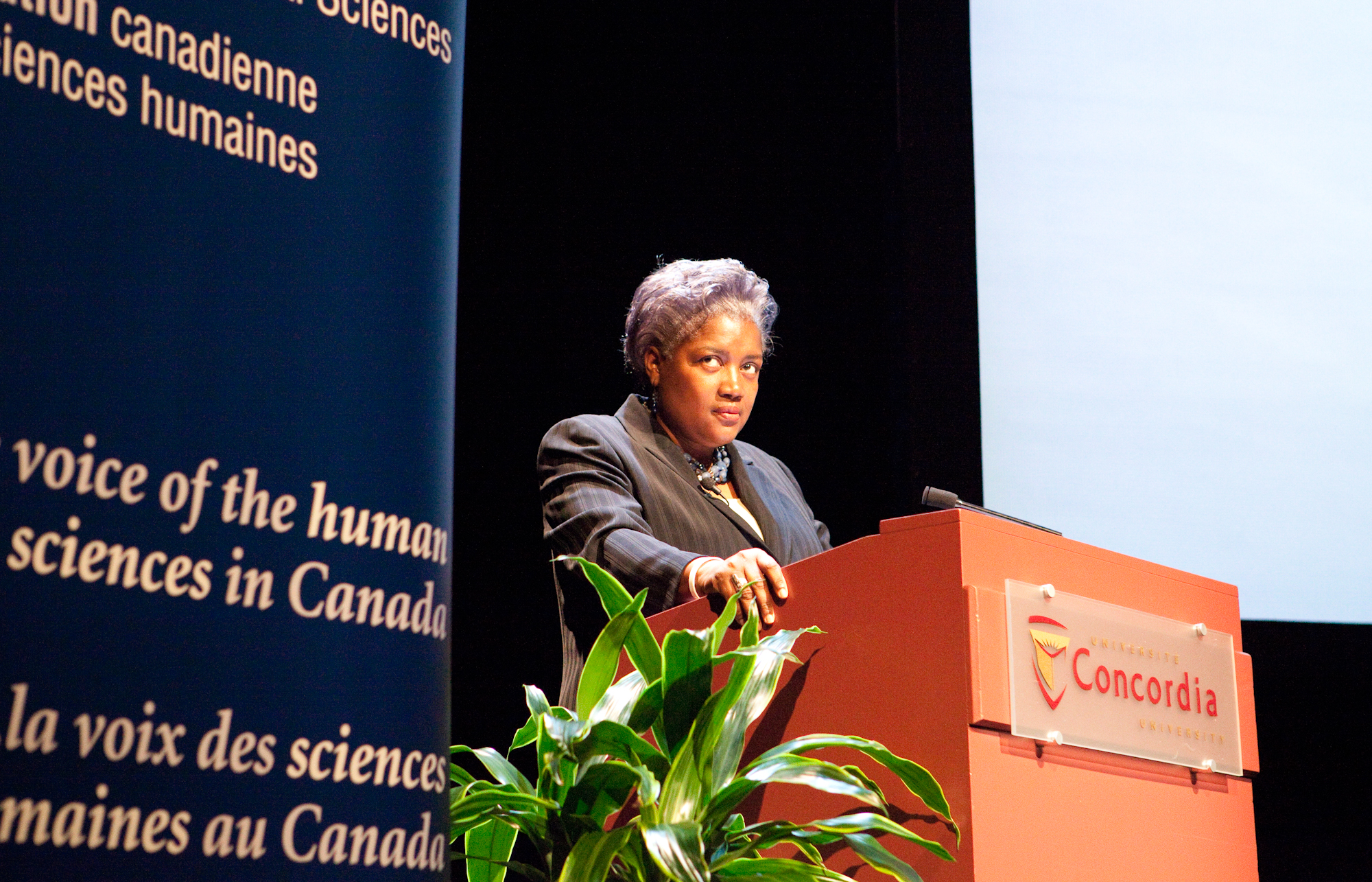This is a horizontally aligned rectangular photograph depicting a poised woman standing at an orange, wood-like podium adorned with a clear acrylic placard that reads "Concordia" in red text, mounted by four silver caps. The woman, a Black individual with short, graying hair, is wearing a black suit with a scarf or large blue necklace underneath. She stands silently with her mouth closed, glancing off to the left as if attentively listening to someone. Behind her is a backdrop comprising a black curtain. To the left of the podium, there is a partially visible banner with gold lettering that states "The Voice of the Human Sciences in Canada" in both English and French, with fragments like "Canadiennes Sciences Humaines" and "Le Voyage des Sciences." Between the banner and the podium, a green fern plant is visible. On the upper right side of the image, a large blank white projector screen is present. The setup signifies a formal event or conference setting, emphasizing the intellectual and academic atmosphere.